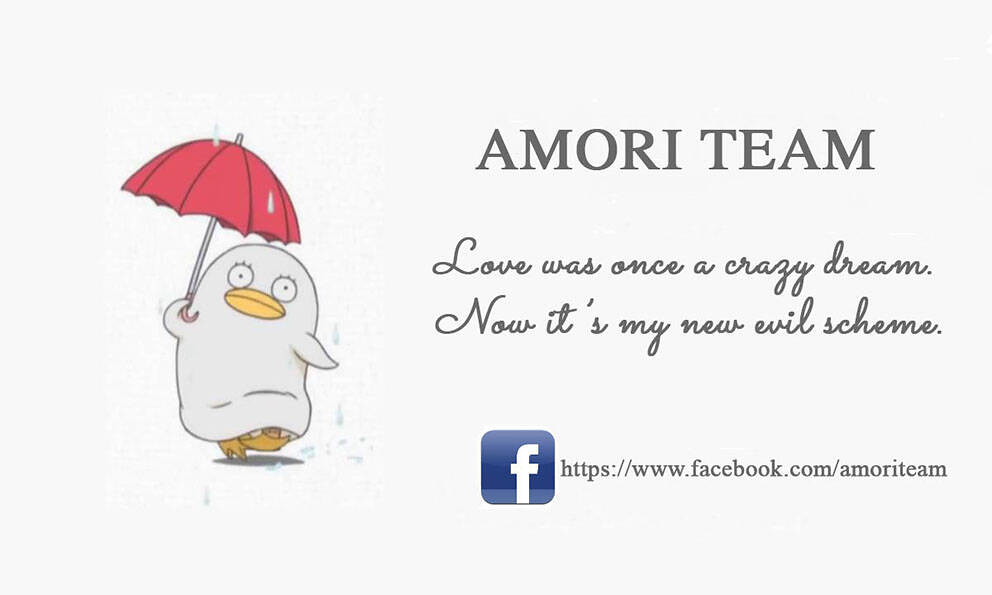This image is a color graphic commonly referred to as a meme or inspirational quote, found on Facebook. The entire graphic is set against a white background, resembling a business card.

On the left side, there's a small, cute drawing of a duck. The duck features big, circular eyes with simple dots and small eyebrows. It has a yellow beak and yellow feet but is otherwise dressed in what appears to be white cloth-like clothing. The duck is holding a red umbrella with a thin stick and a small yellow curve at the bottom, seemingly blocking off rain.

To the right of the duck, the text "AMORITEAM" is displayed prominently in bold, uppercase letters. Below that, written in cursive, is the phrase "Love was once a crazy dream, now it's my new evil scheme." Further down, the Facebook logo (an 'F' on a blue background) is shown next to the web address "https://www.facebook.com/AMORITEAM."